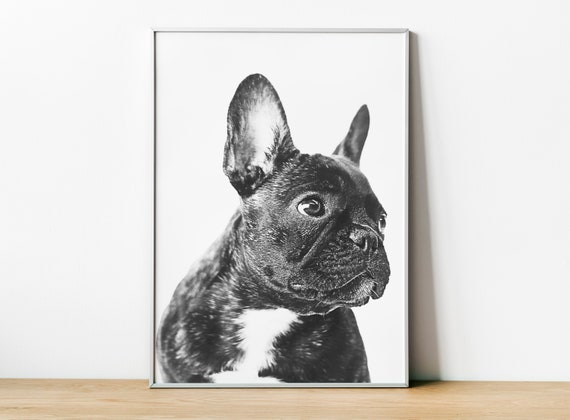The image depicts a photograph of a framed picture of a small French bulldog, positioned against a white wall and resting on a wooden floor. The black and white framed picture, which is centered in the image, features a French bulldog with a mostly black coat, accentuated by a white patch running from its chin down its chest. The dog's large, rounded ears are pricked up, and its expressive, slightly bulging eyes give it a distinctive look. The photograph cuts off just below the dog's torso, leaving its legs unseen. The dog's smushed face, characteristic of French bulldogs and pugs, has shiny details around the nose and visible whiskers protruding from its chin. The frame is thin and metallic, with a small shadow cast to the right where it leans against the wall. Only the top half of the dog is visible, capturing its head and chest in a side-on, turned-to-the-right pose. The simplicity of the white background within the framed picture contrasts with the various shades of black in the dog's fur, highlighting its unique features.